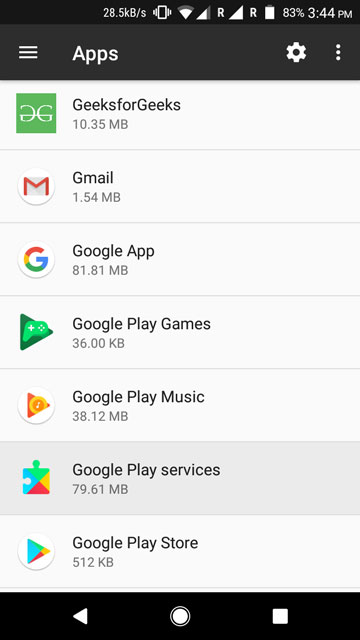This image features a cropped screenshot of a cell phone’s applications page. At the top of the screen, there is a black banner with the word "Apps" displayed in bold white letters on the left. To the right of the word "Apps," there is a white menu icon. Further to the right, on the far right end of the banner, there is a cogwheel icon for settings and another menu icon. 

Below this black banner, the main background of the app display is white. The apps are listed vertically, showing each app's icon, name, and size. Each app icon is positioned to the left, with the app's name just to the right of its icon, and the app size directly below the app's name. 

The first listed app has a green square icon labeled "Geeks for Geeks," and its size is noted as 10.35 megabytes. Below this, the second app is "Gmail," with a size of 1.45 megabytes. Following these, the apps listed are "Google App," "Google Play Games," "Google Play Music," "Google Play Services," and finally, "Google Play Store."

At the very bottom of the screenshot, a black navigation bar displays three standard phone icons: a triangle on the left for returning to the previous page, a circle in the middle for going to the home screen, and a square on the right for accessing recent apps.